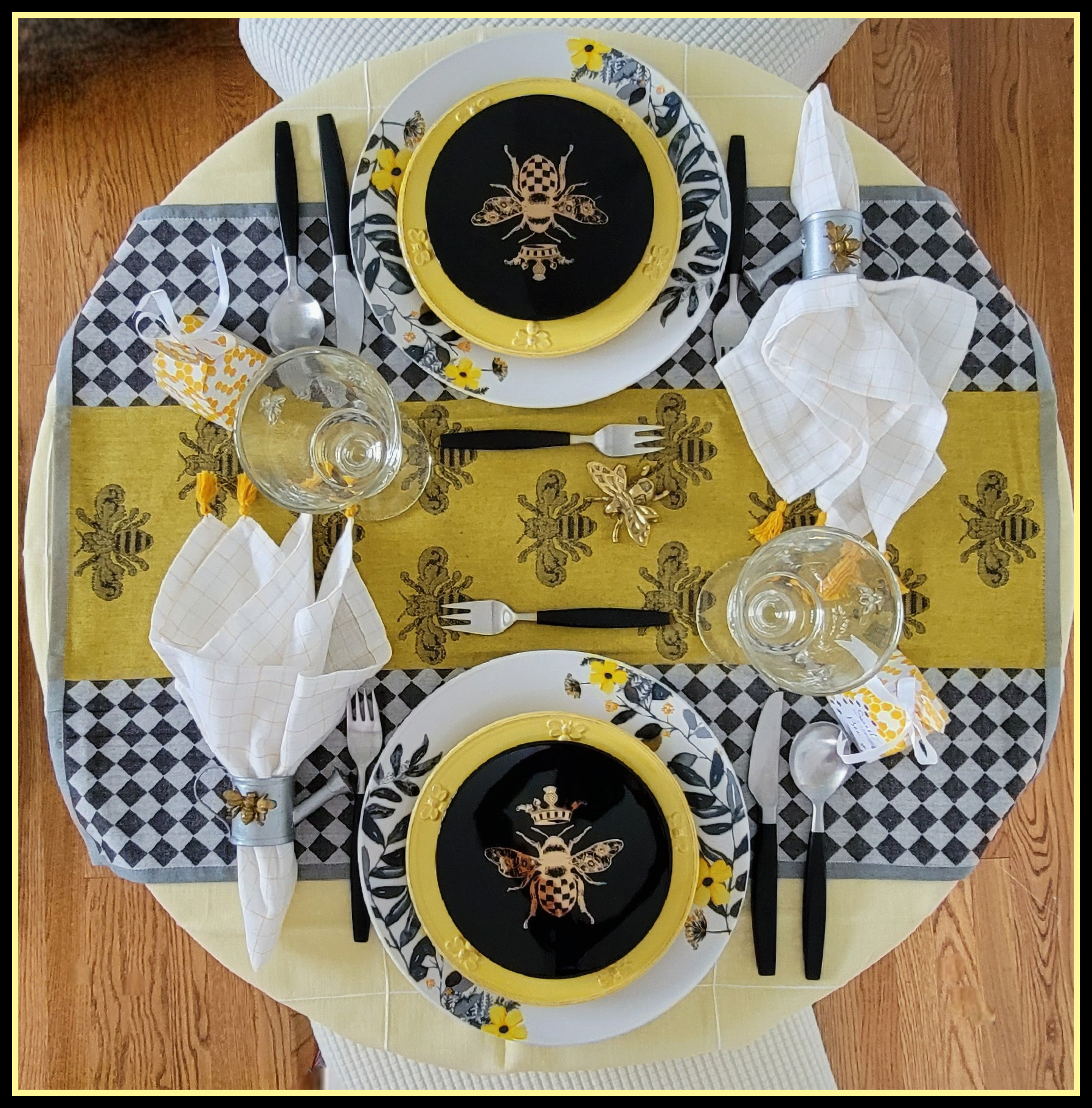This is a detailed overhead photograph of an elegantly arranged round table featuring a sophisticated blend of yellow, black, and white elements. The table, with a brown wooden surface, is adorned with a distinctive tablecloth showcasing a central insect design, framed by gray, golden, and black accents. Surrounding the design are black and gray checkered patterns. In the middle of each setting are two stacked round plates: the bottom plate is primarily white with black and yellow floral patterns, while the top plate or tiny bowl is yellow, featuring a bumblebee in the center against a black background.

Accompanying the plates are pieces of silverware, which include knives, spoons, and forks with black handles and silver tips. Each place setting also features a white napkin positioned to the side, and an arrangement of forks placed strategically on both sides of the plates. To complete the arrangement, two clear wine glasses are strategically positioned—one by the bottom plate and another by the top plate. Additionally, there's a small yellow favor bag adorned with a white bow, hinting at a festive or celebratory occasion.

This meticulous table setting exudes a harmonious color scheme, with yellow elements beautifully contrasted against the black, white, and gray details, creating an inviting and aesthetically pleasing dining experience.